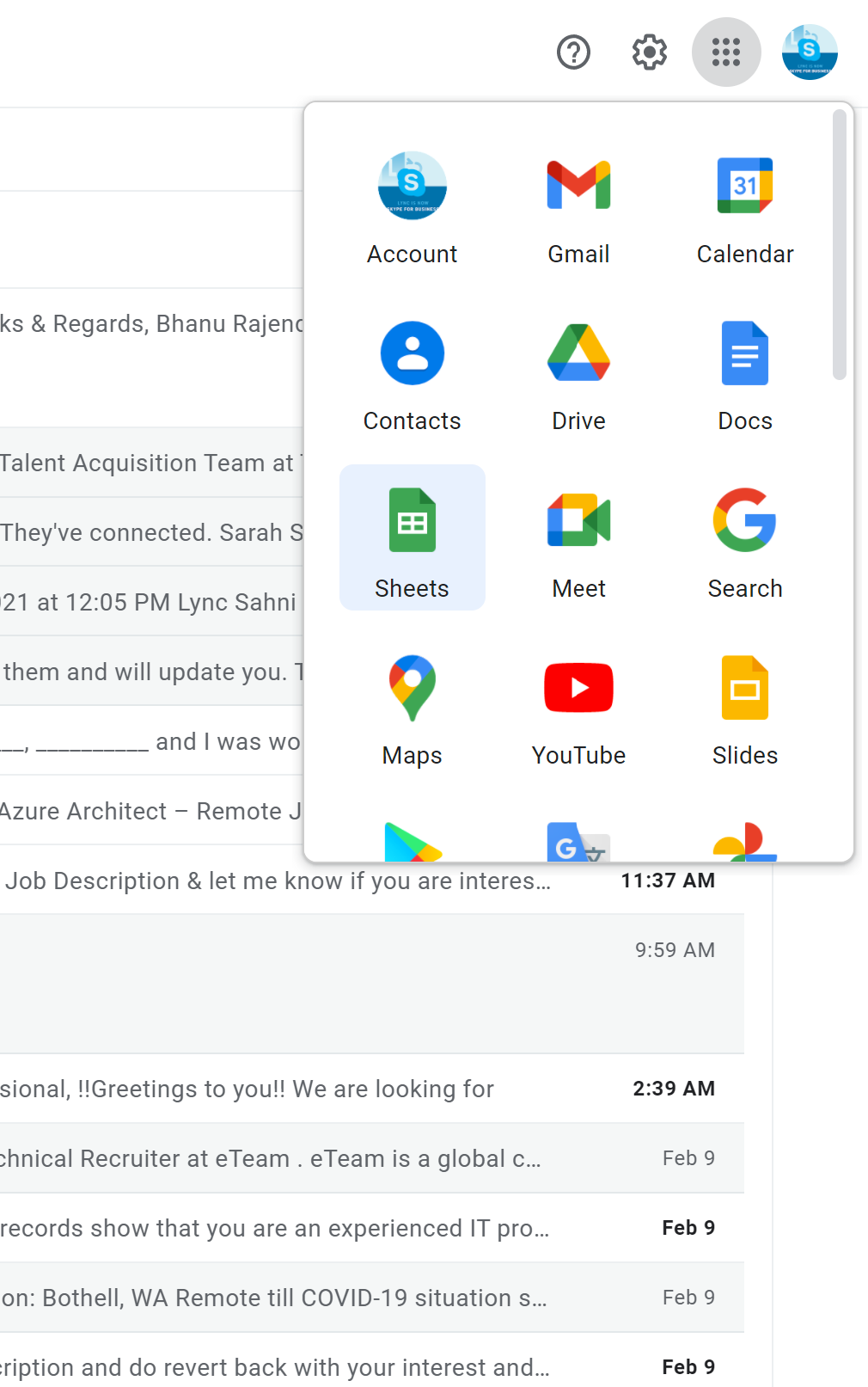The image showcases a partial view of an email interface, where a pop-up window displaying various Google apps is open. In the pop-up, the apps are organized into a grid with three columns and five rows, although the bottom row is partially cut off, concealing the names of three apps. The visible apps are presented in the following order:

1. **First Row:** Account, Gmail, Calendar
2. **Second Row:** Contacts, Drive, Docs
3. **Third Row:** Sheets, Meet, Search
4. **Fourth Row:** Maps, YouTube, Slides

Each app is represented with its corresponding icon. The main email interface is partially visible in the background, revealing only the far right edge. Here, a snippet of an email subject line and either the time or date of when the email was sent can be seen.